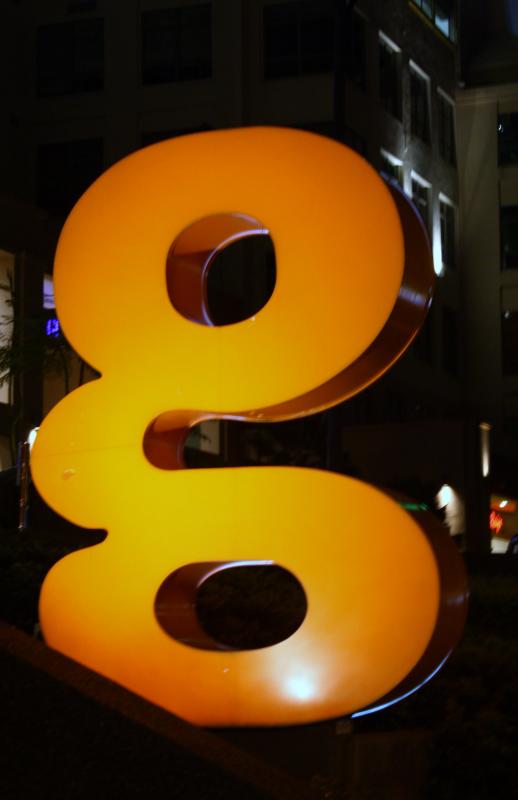This detailed color photograph captures a nighttime or early morning scene featuring a vivid, stylized 3D sculpture resembling the letter "G." The sculpture is predominantly orange, with lighter, almost yellow hues in its middle section due to the lighting. The "G" consists of a top and bottom circular part connected by a semicircular squiggle, creating a uniquely stylized lowercase 'g' form. The background reveals a few buildings, including a taller structure approximately four to five stories high and a shorter adjacent one, all dimly lit against the dark sky. Slightly obscured in the bottom-left corner of the image, there is an object casting a shadow on the "G." Additionally, a faint blue neon sign is visible behind the sculpture, contributing to the atmospheric lighting. A tree is also discernible to the left side of the photo, further emphasizing the outdoor setting. The contrasting illumination and architectural elements bring a distinctive charm to this intriguing urban snapshot.